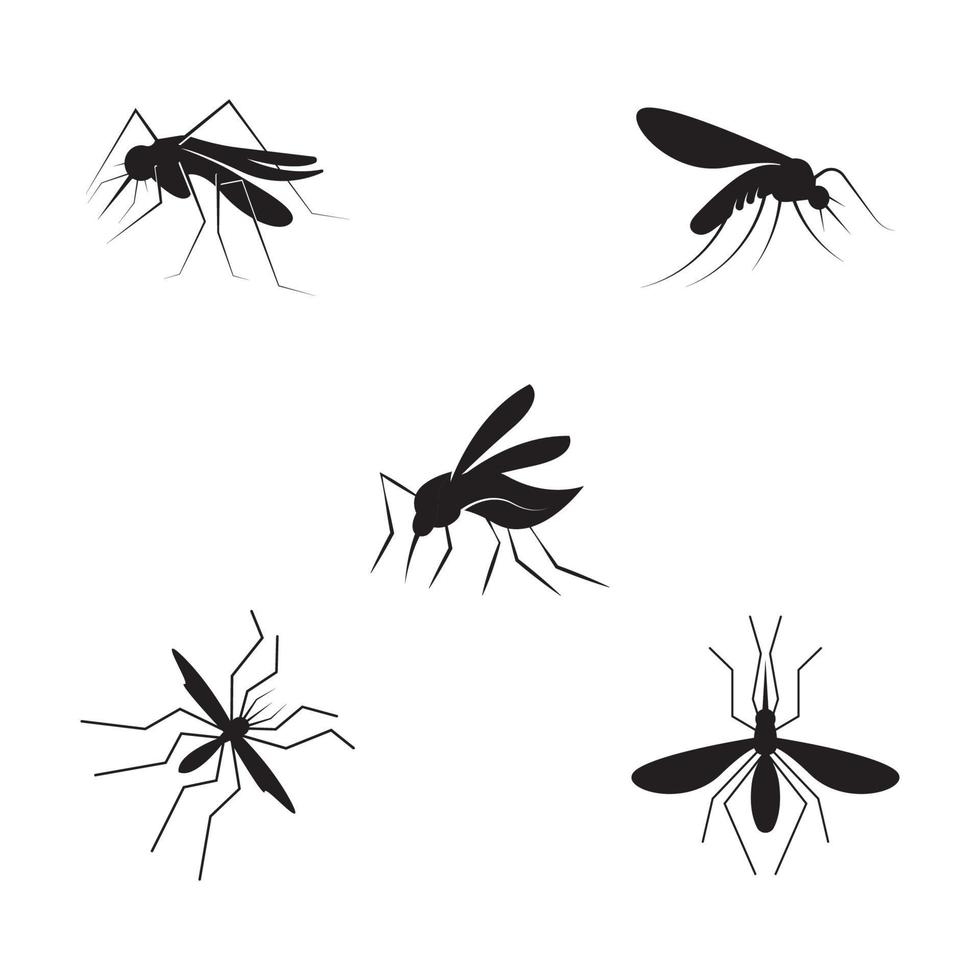The image features five black, clip art-style mosquito icons on a stark white background, arranged with one in each corner and one in the center. In the upper left corner, there is a detailed side-view mosquito facing left, displaying one wing and several legs. The upper right corner has another side-view mosquito, this time facing right, also showing one wing and multiple legs. The center mosquito is a side view with its body angled towards the viewer, allowing visibility of both wings and all legs. The lower left mosquito is depicted from above, showcasing both wings, all legs, and its antennae. Lastly, the lower right mosquito is also shown from an overhead view, similar to the lower left but a bit more rounded in shape. All mosquitoes vary slightly in depiction but share the common elements of wings and long legs, highlighting different facets of their forms in the simplified, black silhouette style.